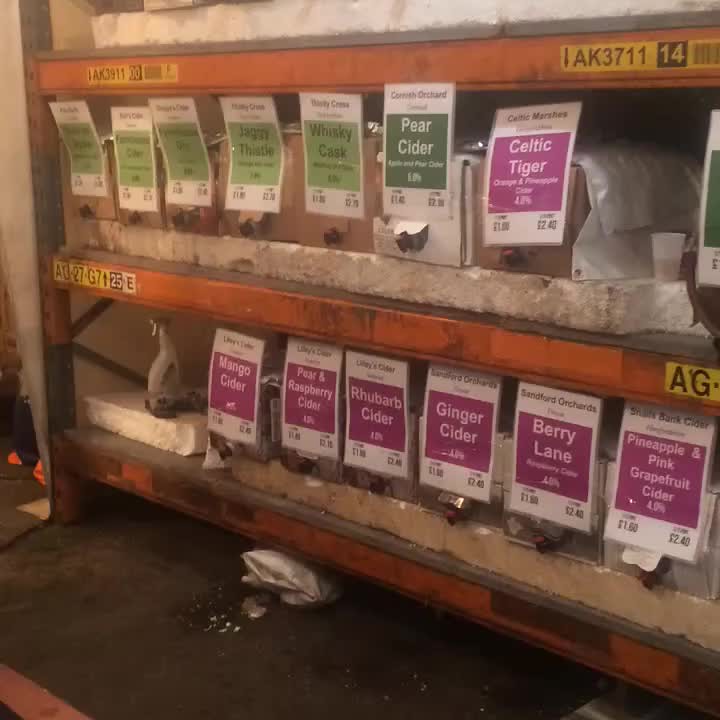In this image, we observe a heavily used, industrial-style metal shelving unit that has an orange front and a silver top, both of which are chipped and dirty. The shelving unit has three rows, although the top row is not visible in the photograph. The shelves are standing on a grimy concrete floor and are supported on the right side by a prominent steel bar.

The middle row is stocked with rectangular boxes, each adorned with large white tags. The first four tags from the left have light green centers with dark green writing, while the fifth tag has a dark green square with white text reading "Parasiter," and the sixth tag has a purple square with white text reading "Celtic Tiger." Further to the right, the boxes progressively move closer to the camera.

The bottom shelf, which is close to the floor, also displays boxes labeled with various cider types, including mango cider, pear and raspberry cider, rhubarb cider, ginger cider, berry lane, pineapple and pink grapefruit cider, as well as pear cider and celtic cider. Additionally, there's a small spray bottle, presumably for cleaning, located at the far left.

The overall scene suggests a rough, utilitarian storage unit filled with assorted cider boxes, some of which have spouts for dispensing.